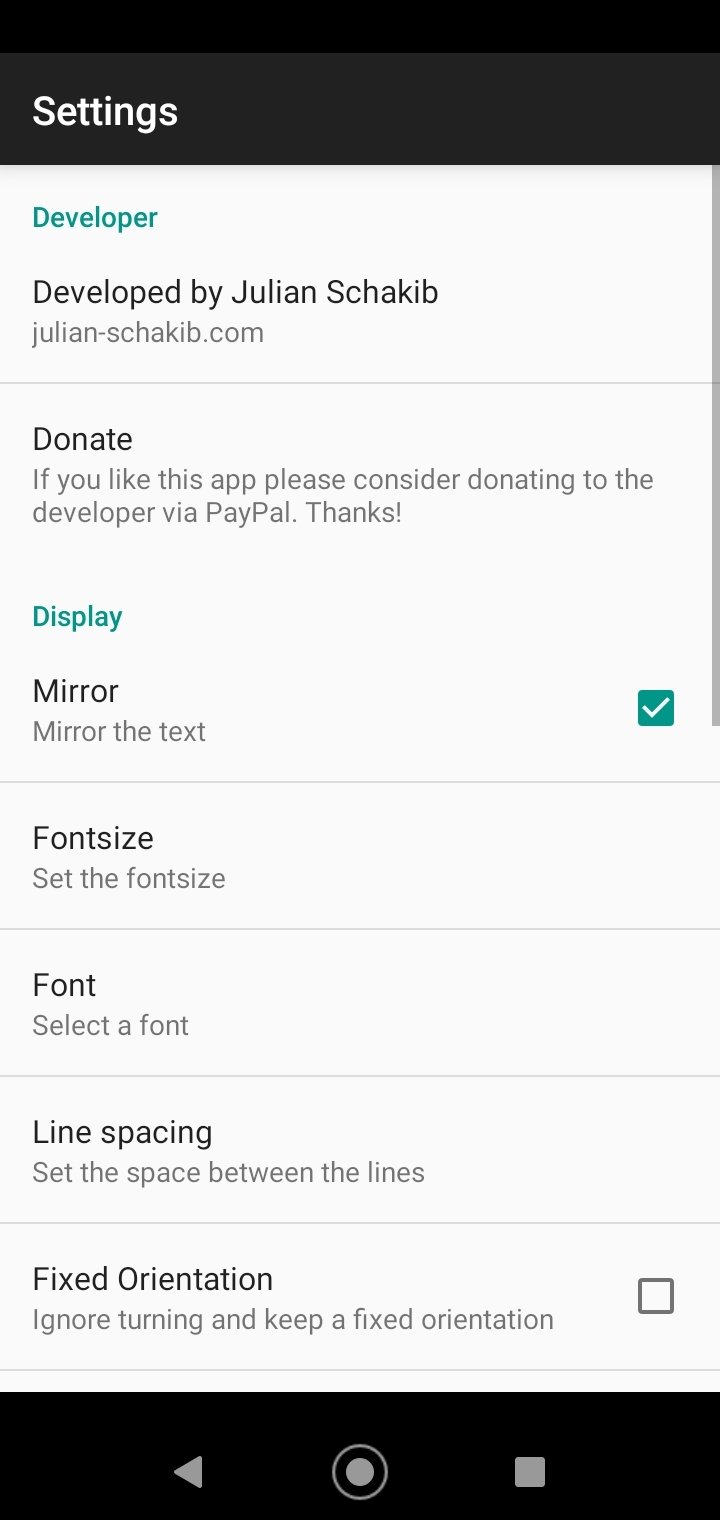The image depicts the settings page of a mobile device. The top part of the screen features a thin black bar, followed by a thicker bar in a brownish-black color. On the left-hand side of this thicker bar, the word "Settings" is prominently displayed in white font, with the 'S' capitalized.

Below this bar, the background transitions to white, and the page is divided into six distinct sections aligned vertically. The sections are as follows:

1. **Developer**: 
    - Subtitle: "Developed by Julian Schakib"
    - Additional information: "julianminesignschakib.com"

2. **Donate**:
    - Instruction: "If you like this app, please consider donating to the developer via PayPal. Thanks!"

3. **Display and Mirror**:
    - Details: This section includes the text "Mirror" followed by a checkbox, which is currently checked.